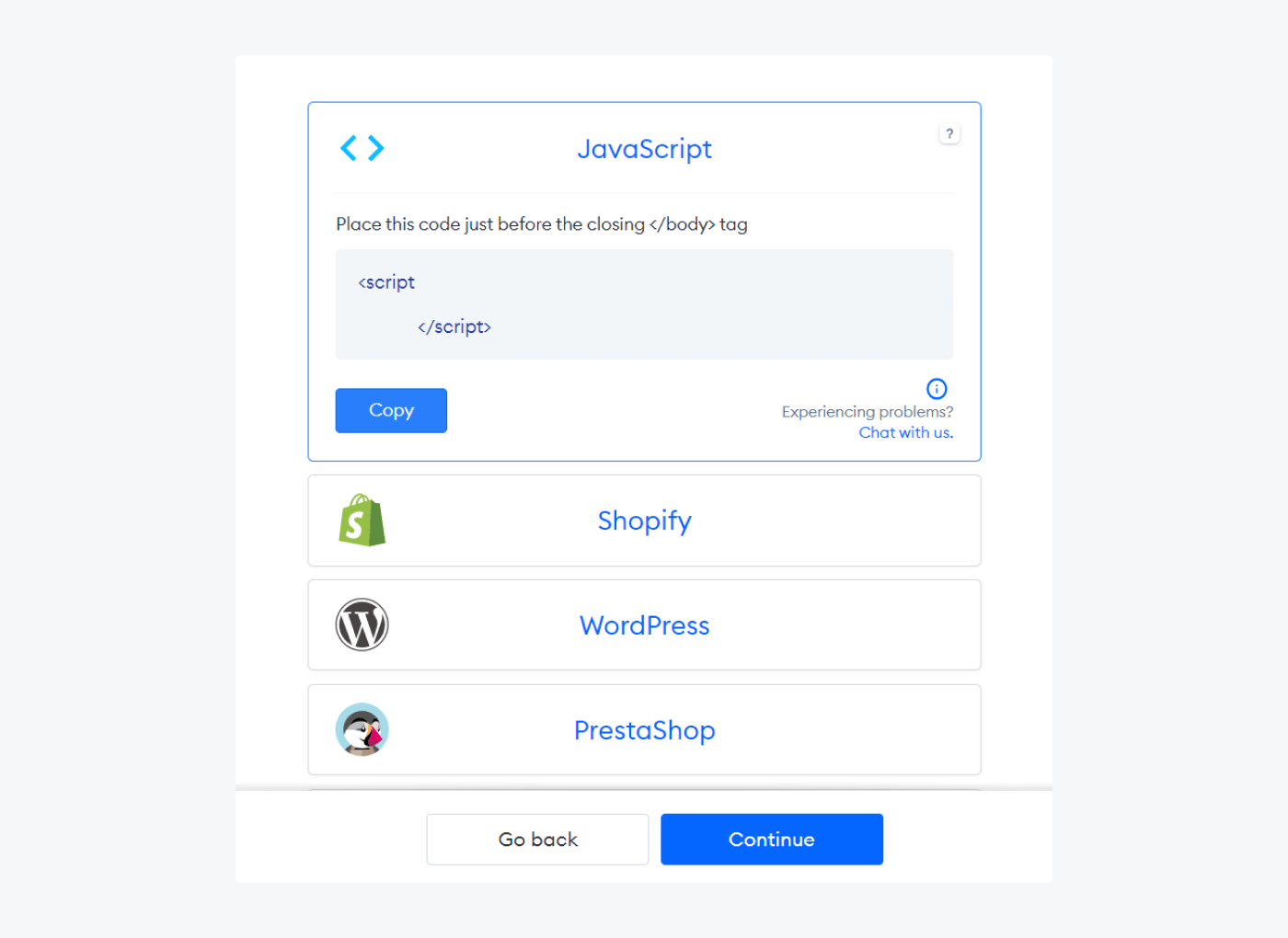A detailed screenshot of a coding interface on a website with a clean and user-friendly design. The background is entirely white, contributing to the interface's neat appearance. At the top, in prominent font, is the heading "JavaScript," flanked by two bracket symbols resembling Pac-Man mouths facing each other. 

In the top right corner of the header, there's a small blue box containing a question mark, likely indicating additional help or information. Directly beneath the main "JavaScript" heading, also within the blue box, is a line of black text instructing the user to "place this code just before the closing </body> tag."

Below this instruction is a code insertion box with placeholder text, showing an opening and closing script tag: "<script></script>." Adjacent to the insertion box is a blue "Copy" button for easy copying of the script code.

Further down, there is a support link for iOS users experiencing issues, labeled "chat with us." 

The interface also features three different platform options, each with their respective logos: Shopify, WordPress, and PrestaShop (depicted with a penguin logo). 

At the bottom of the screenshot, two blue buttons are available for navigation: "Go Back" and "Continue."